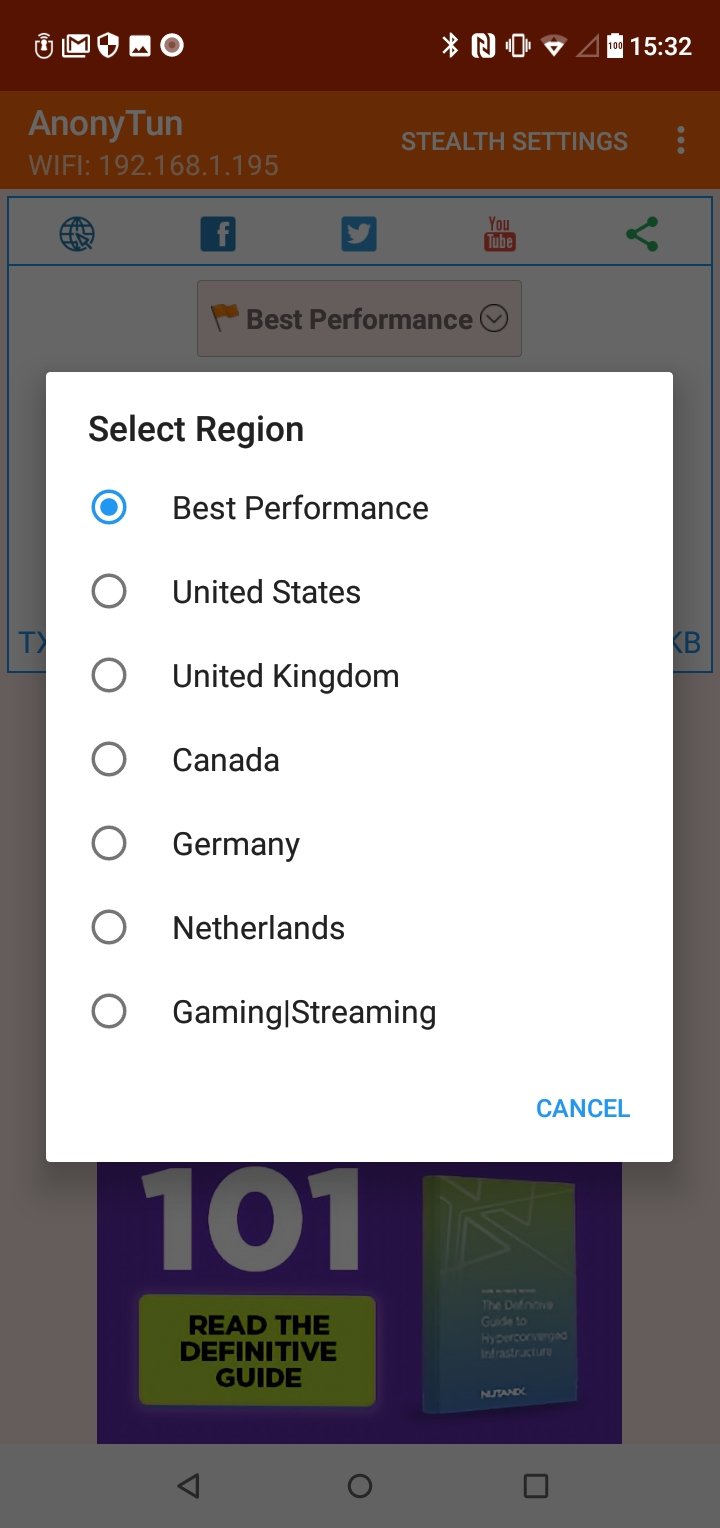This image is a detailed screenshot from a smartphone. The top border features a dark red, almost maroon, color. In the top right corner, the time is displayed in white font as 15:32, indicating the use of the 24-hour clock format. The battery icon shows nearly full charge, accompanied by wireless connection and Wi-Fi icons. Additionally, there's an icon indicating the phone is on mute.

Beneath the top header, the website content appears grayed out due to a white pop-up box dominating the center of the screen. Despite the gray overlay, the top header of the webpage is visible with an orange background displaying "ANONYTUN" in white font, and "Stealth Settings" on the right side.

The white pop-up box in the middle of the screen contains gray text that reads "Select Region". At the top, "Best Performance" is shown with a selected blue-outlined circle, indicating it as the chosen option. Below this, unselected options listed with gray circles include United States, United Kingdom, Canada, Germany, Netherlands, Gaming, and Streaming. 

In the lower right-hand corner of the pop-up box, "Cancel" is written in blue font.